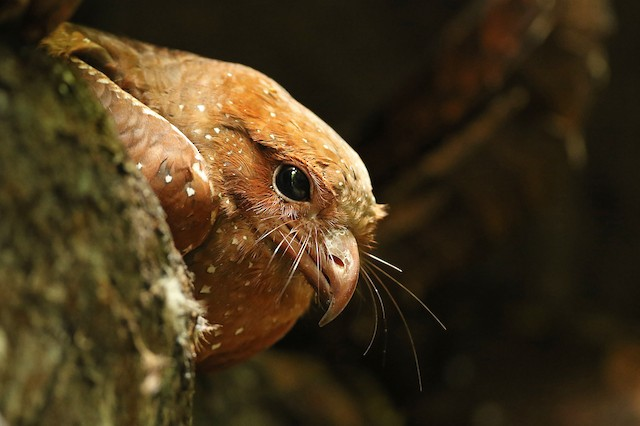This close-up photograph captures a serene moment featuring an orange bird perched on what appears to be a rough tree trunk or stone with hints of moss. The bird, predominantly shades of orange with subtle transitions into brown, white, and reddish tones, is positioned on the left side of the landscape-oriented image. Its elegant profile reveals a slightly curved, orange beak, dark round eyes, and distinctive whisker-like feathers extending from either side of its beak. Its wings, tucked in close to its body, display a scattered pattern of diamond-like white speckles. The background, occupying the right third of the photo, is artfully blurred with an array of dark brown, black, and red hues, suggesting out-of-focus foliage. This blurred backdrop accentuates the fine details of the bird's vivid plumage and curious gaze directed to the right.